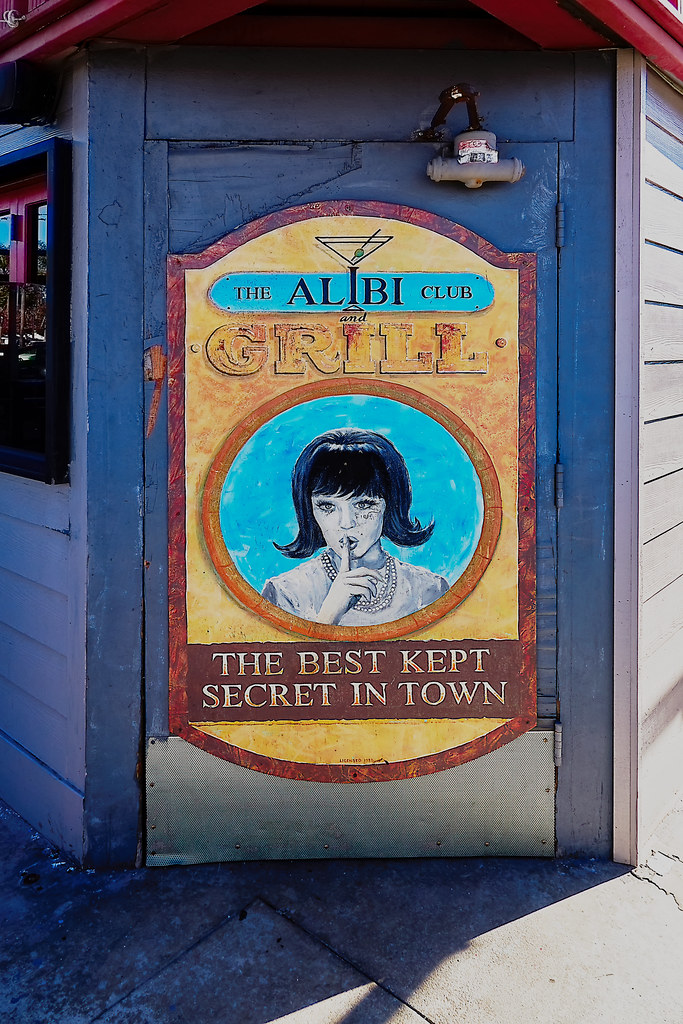The photograph captures the rustic charm of a weathered white building with red-trimmed roof eaves and a medium faded blue door that stands prominently. This building, possibly a shack, houses the Alibi Club and Grill, known as "the best-kept secret in town." A striking yellow sign, rectangular in shape with brown accents, adorns the door. The central feature of the sign is an illustration of a young woman with a 60s mod haircut—complete with flipped shoulder-length hair and bangs—wearing a strand of pearls. She holds a finger to her lips in a 'shh' gesture, emphasizing the club's secretive allure. Her image is enclosed within a circular, aqua blue background. Above her, "The Alibi Club" is inscribed in black letters, flanked by objects like a martini glass cleverly integrated into the lettering. Beneath her, the banner declares "the best-kept secret in town" in yellow letters, adding to the playful and inviting mystery of this unique venue.